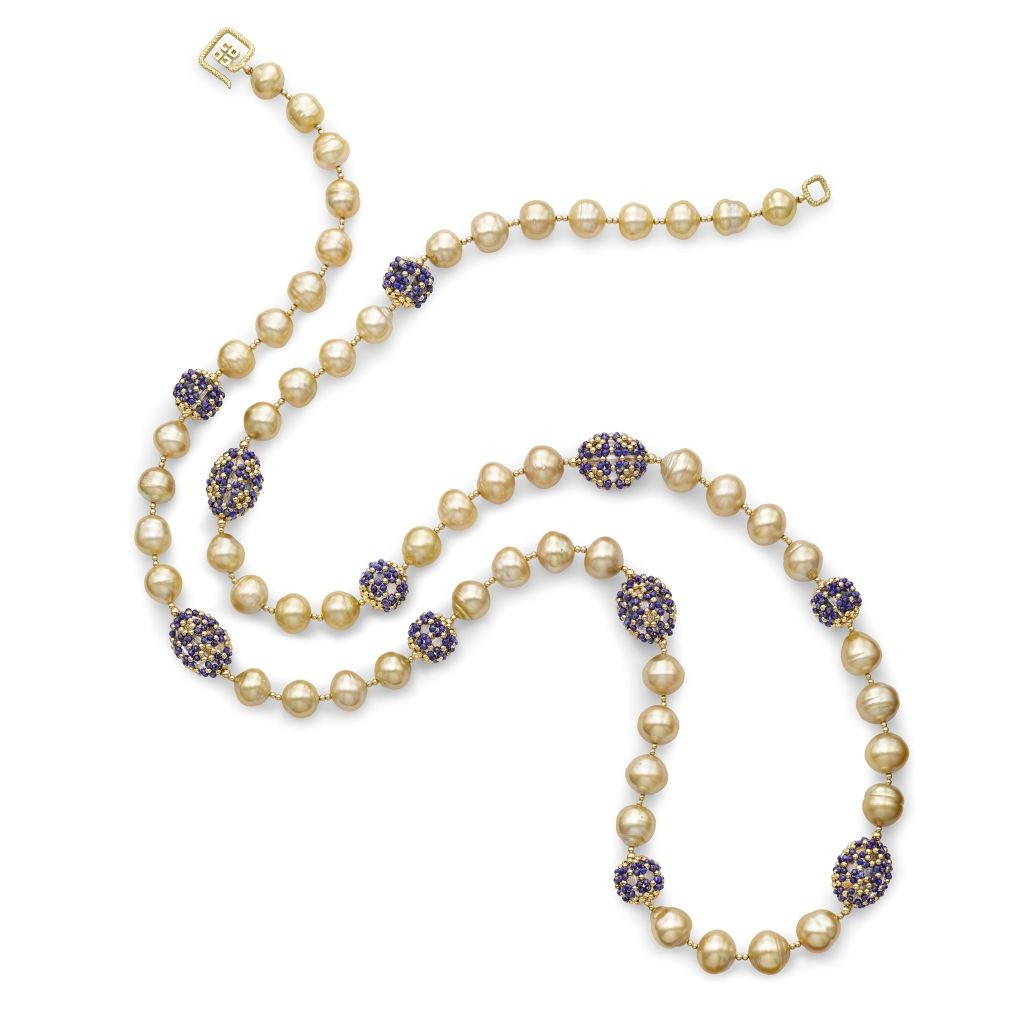This image showcases an intricately designed pearl necklace set against a pristine white background. The necklace, laying out in an elegant S-shaped pattern, features a gold chain and clasps. Each clasp includes a square gold piece for fastening, adding a touch of luxury to its design. The main body of the necklace is composed of a repeating pattern: groups of off-white to lightly golden round beads, interspersed with unique purple and gold decorative beads. Specifically, the design alternates between clusters of eight white round beads, followed by a single blue and gold bead, then four white round beads, followed by another blue and gold bead. The decorative beads vary slightly in shape, ranging from somewhat oval to circular, further enhancing the necklace's intricate charm. This detailed arrangement exemplifies a blend of classic elegance and contemporary design elements.